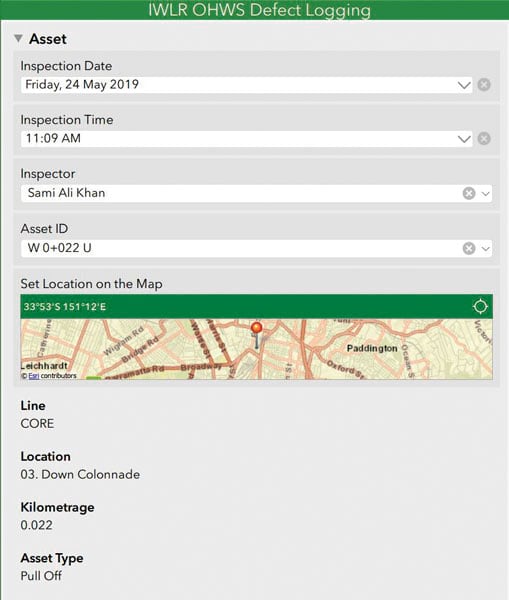The image features a detailed interface for defect logging in the "IWLR OHWS" system. Across the top is a green strip with white text, reading "IWLR OHWS Defect Logging." On the left, it lists "Asset," and next to it is the "Inspect Date," which has a dropdown menu and displays Friday, 24 May 2019. To the right side of this field, there is a circular 'X' button. Below, the "Inspect Time" is noted as 11:09 AM, also accompanied by a dropdown and an 'X' button.

Next, the inspector's name is provided as "Sammy ALI KHAN," with 'X' and dropdown options available. The "Asset ID" is indicated as "WO022U" (or possibly "W0022U"), again with an 'X' and dropdown. Underneath, the "Asset Location on the Map" is specified with coordinates "33 degrees 53' South, 151 degrees 12' East," displayed in white font on a green banner that spans the top of the map.

There is a pin on the map illustrating the asset location. Below the map, the text mentions "Line: core," "Location: 03 point," and further corrects "Colonnade." Lastly, the "Kilometric" position is recorded as "0.022" and the "Asset Type" is specified as "Pull Off."